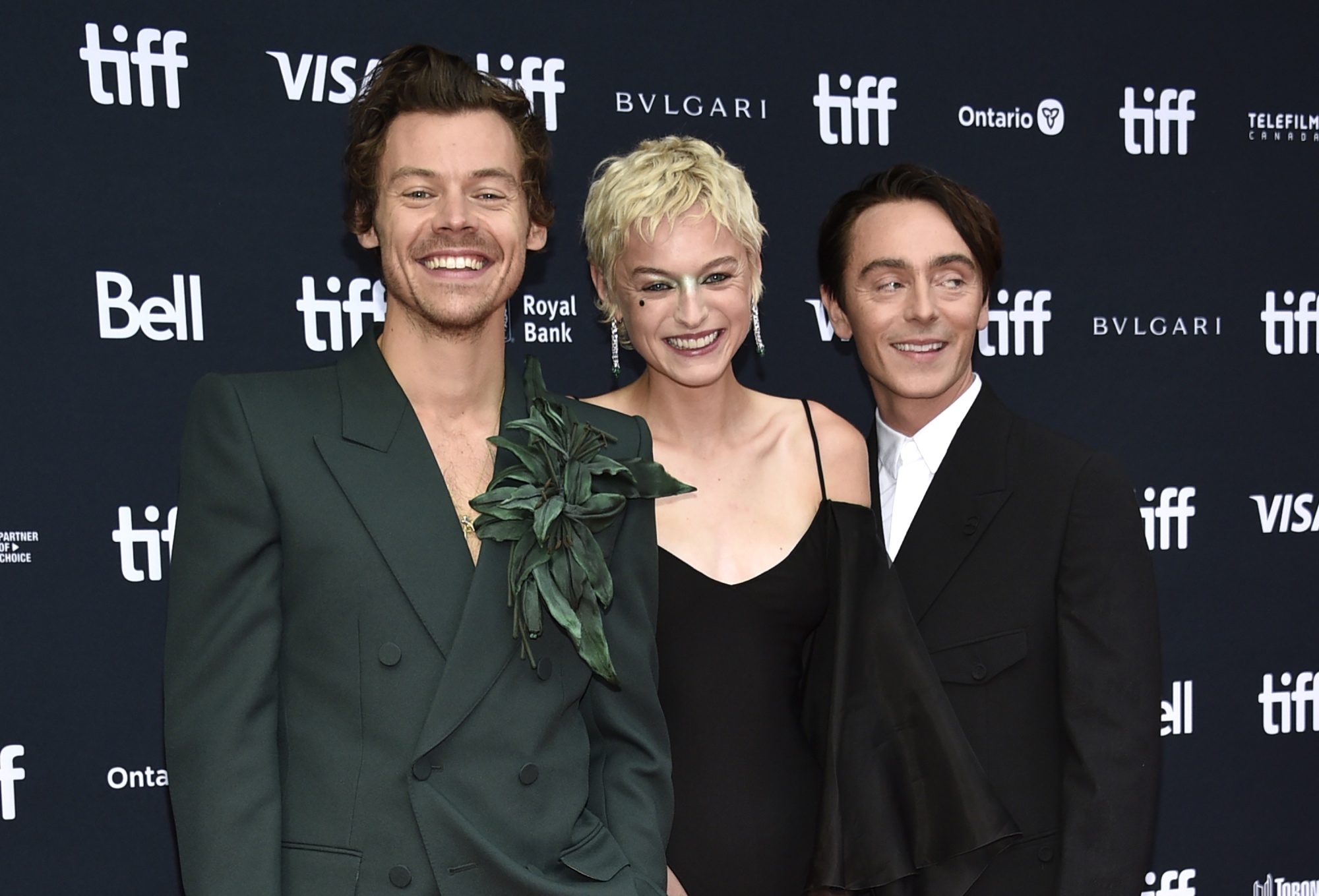In this premier red carpet photograph taken in front of a blue backdrop adorned with white logos reading TIFF, Visa, Bulgari, Ontario, and Bell, three celebrities are standing side by side. On the left is Harry Styles, grinning at the camera in a dark green suit adorned with a floral pin on his lapel. His brown hair is short and neatly styled. In the center is Emma Corrin, wearing a black sleeveless dress with tiny spaghetti straps. Her short blonde hair complements her silvery long earrings, and she too is smiling warmly at the camera. To the right stands David Dawson, slightly shorter than the others, dressed in a black suit with a white shirt buttoned up to the neck. His brownish-black hair is combed over to the left, and he is looking off to the right with a smile. The trio's elegant attire and poised smiles make for a captivating image against the backdrop of prominent brand logos.